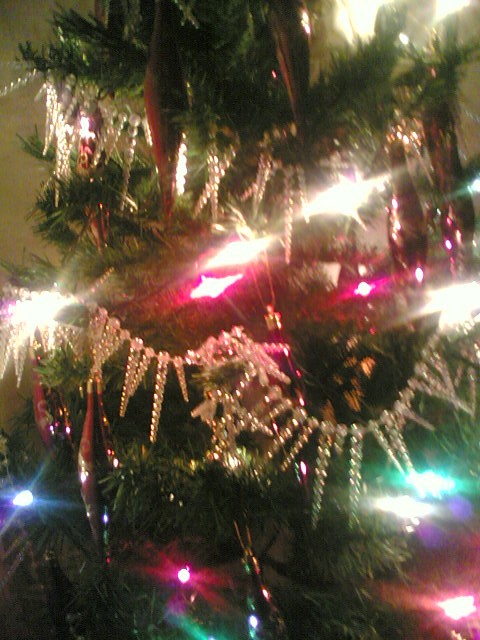In this slightly blurred close-up portrait photograph of an artificial Christmas tree, the dark green pine needles create a lush backdrop for an array of festive decorations. The tree is adorned with multiple garlands of decorative ropes, each strung with small, silver beads designed in triangular shapes. These garlands cascade around the tree, complementing the various strings of brightly colored lights. The lights, which include blue, purple, red, pink, green, and white, appear as diamond-shaped smudges due to the photograph's blur, adding an ethereal glow to the scene. Additional highlights include slender, gold icicle-like ornaments, as well as pointy, elongated decorations with round centers, hanging delicately from the branches. The overall effect is a sparkling, whimsical display, albeit viewed through an intentionally softened lens.